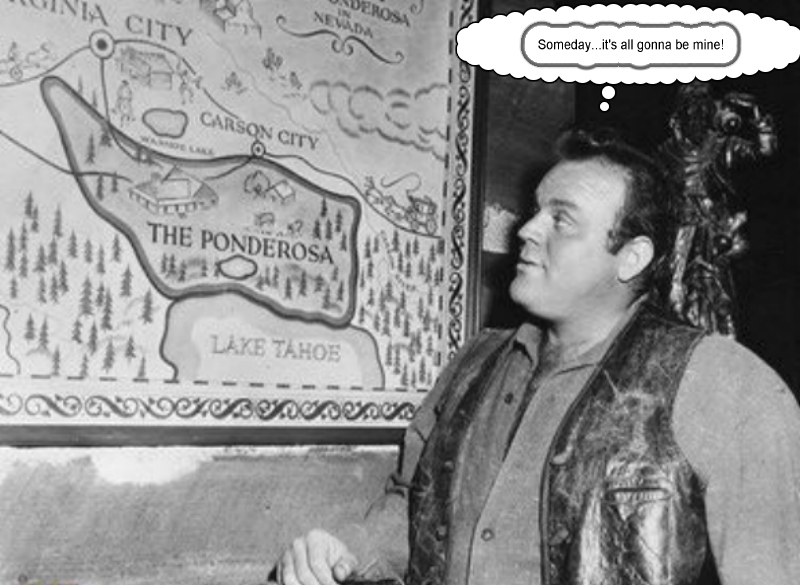This detailed black-and-white photograph from the 1960s TV show "Bonanza" features the character Hoss standing on the right-hand side. Hoss, clad in his signature button-down shirt and leather vest, gazes intently at a large wall map of the Ponderosa. Floating above Hoss's head is a cartoon-like thought bubble that reads, "Someday it's all going to be mine." The map prominently displays key locations such as the Ponderosa Ranch, Lake Tahoe, Carson City, and Virginia City. The Ponderosa, characterized by its lush landscape with trees, a pond, and various buildings, stretches northward from Carson City. This map, a familiar visual from the show's opening sequence, highlights the expansive territory of the Ponderosa Ranch, rooting it firmly in the scenic backdrop of Nevada.